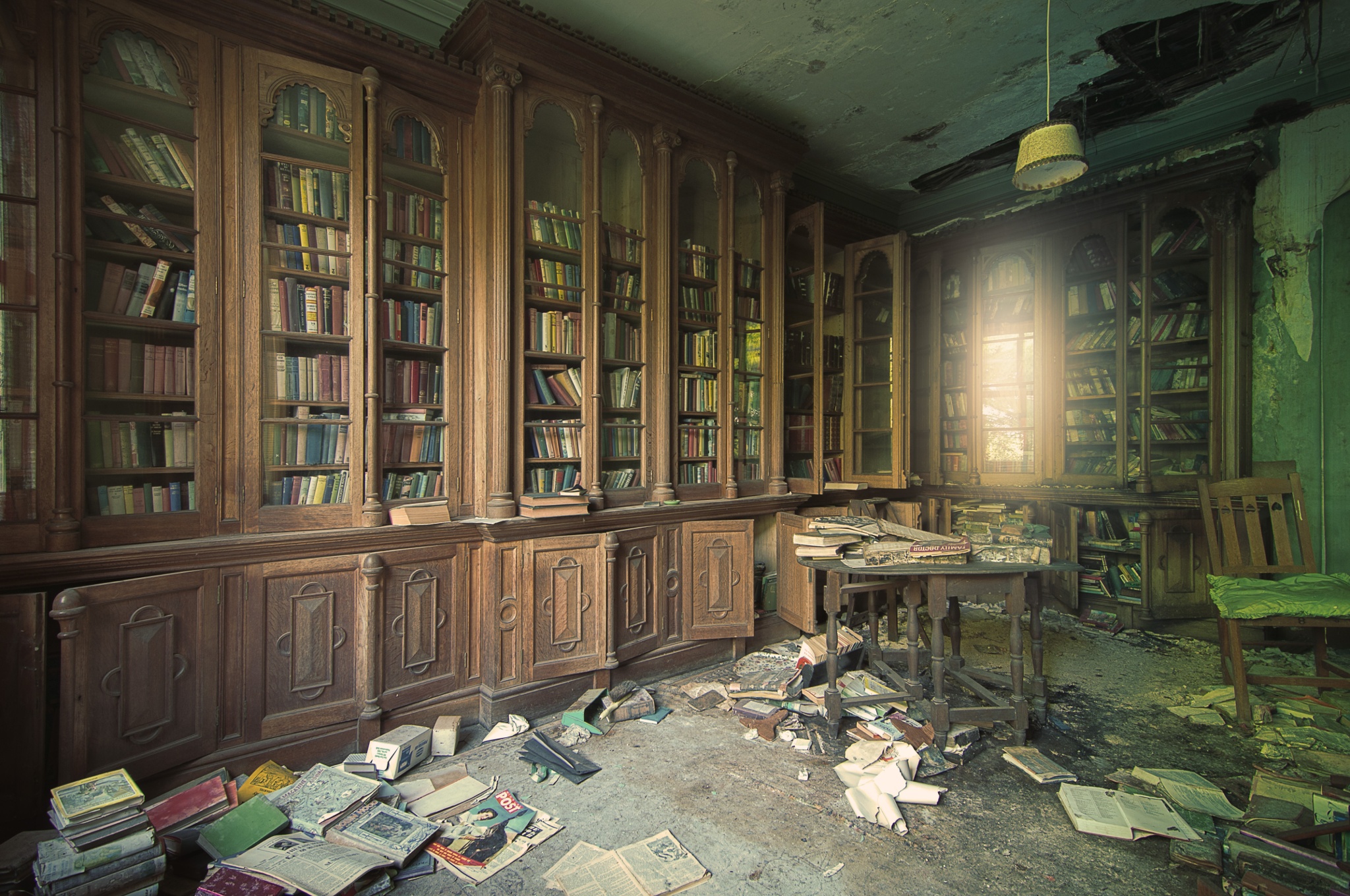The photograph depicts an abandoned, dilapidated library within an old estate. The room is characterized by its derelict condition, with significant details adding to its depiction of neglect and ruin. The left and right walls are lined with tall wooden bookcases, their upper sections enclosed by glass-paned doors revealing shelves crammed with books, while the lower sections feature smaller cupboards, some of which are open and exposing more books and magazines. The floor is heavily worn and scattered with torn and water-damaged books. At the center of the room, a wooden table, laden with books, appears unstable and slouching. The ceiling has large holes, with wooden debris fallen to the floor, and a disused light fixture dangles precariously. The peeling wallpaper on the far right wall and the rotting floorboards further emphasize the space's abandonment. A bright light shines on the bookcase against the back right wall, likely reflecting sunlight from an unseen window, adding a stark contrast to the room's general decay.